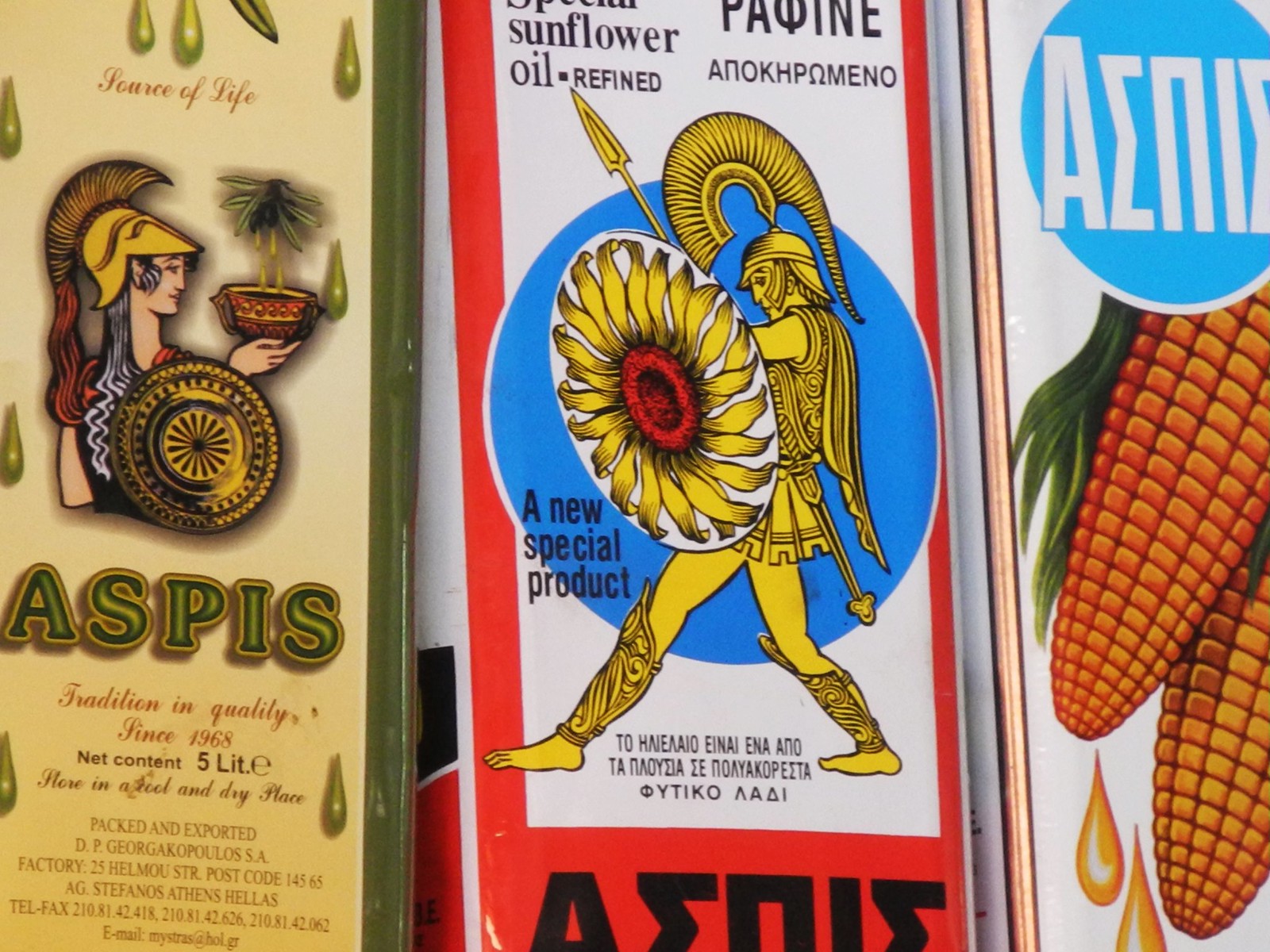This image showcases a close-up view of three vintage-style oil bottles, aligned closely with no visible spacing between them. The background is indiscernible, making the focus solely on the bottles. 

On the left, there's a five-liter bottle of olive oil, characterized by its green-bordered label and green drippings. The label features a woman in Roman attire holding a shield and a potted plant, and it bears inscriptions including "aspis," "tradition and quality," and "since 1968."

The middle bottle contains sunflower oil, distinguished by a red, black, and white label. It prominently depicts a Greek warrior with a sunflower-adorned shield, and it reads "sunflower oil refined" and "a new special product."

To the right, the bottle of corn oil is depicted with white labeling, showing images of corn on the cob with yellow oil droplets trickling off. The color palette across the bottles includes green, tan, yellow, red, black, blue, light blue, orange, and white, suggesting a setting likely inside a grocery store.